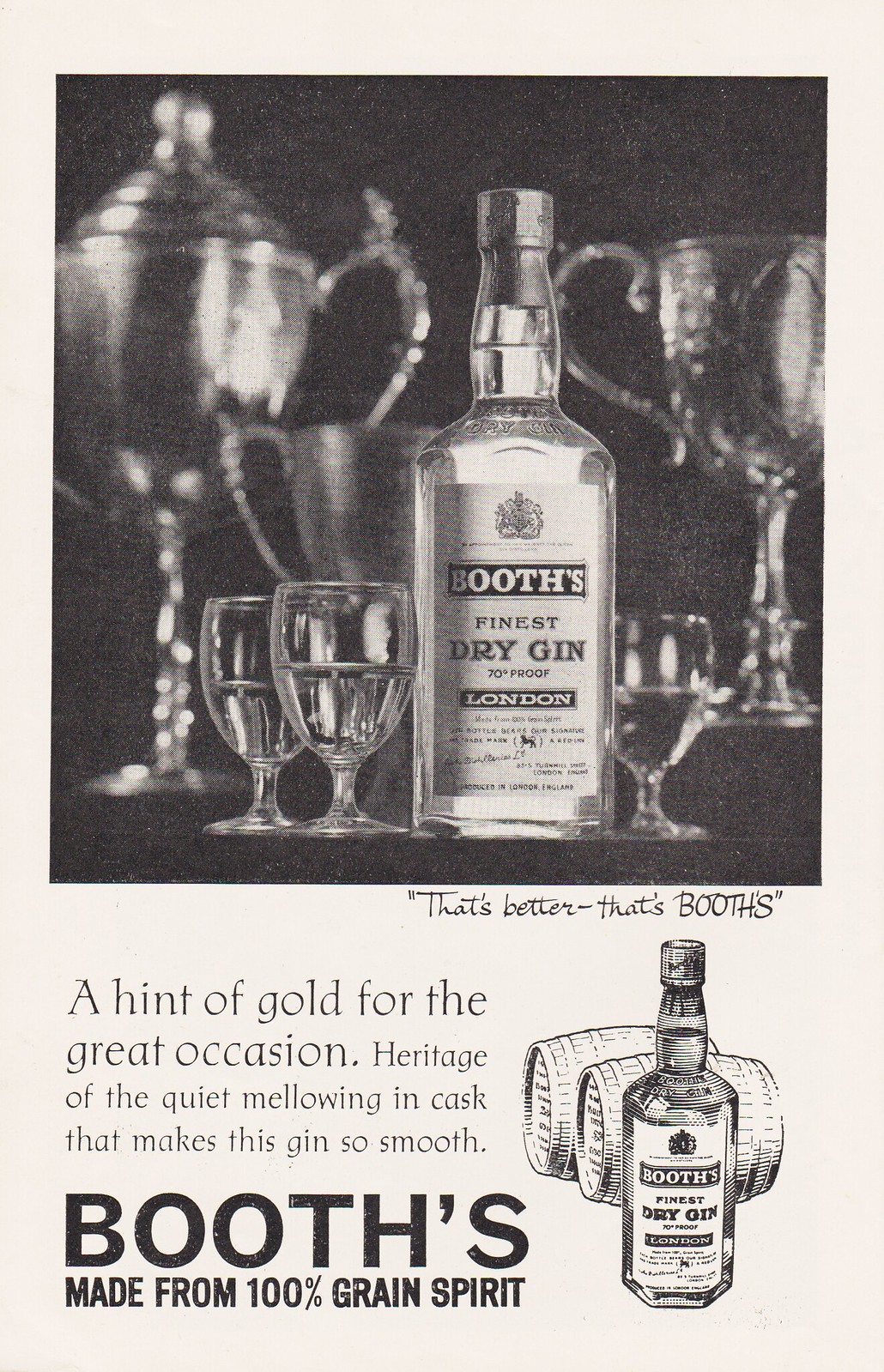This black-and-white advertisement for Booth's Finest Dry Gin highlights a blend of photographic and hand-drawn elements to create a luxurious and heritage-rich image. The centerpiece is a detailed photograph of a bottle labeled "Booth's Finest Dry Gin, London," surrounded by three partially filled glasses. Behind the bottle, two elegant, metallic goblets, possibly silver, stand tall, accompanied by a smaller cup. The background is dark, accentuating the metallic luster of the chalices and the clarity of the gin bottle.

Below the photograph, the poster features the tagline: "That's better, that's Booth's." Continuing downward, the ad transitions into a hand-drawn section depicting a bottle of Booth's Dry Gin flanked by two oak barrels, emphasizing the traditional aging process that contributes to its smoothness. The caption reads, "A hint of gold for the great occasion. Heritage of the quiet mellowing in cask that makes this gin so smooth. Booth's, made from 100% grain spirit." This blend of visual and textual elements exemplifies a sophisticated appreciation for quality and tradition.